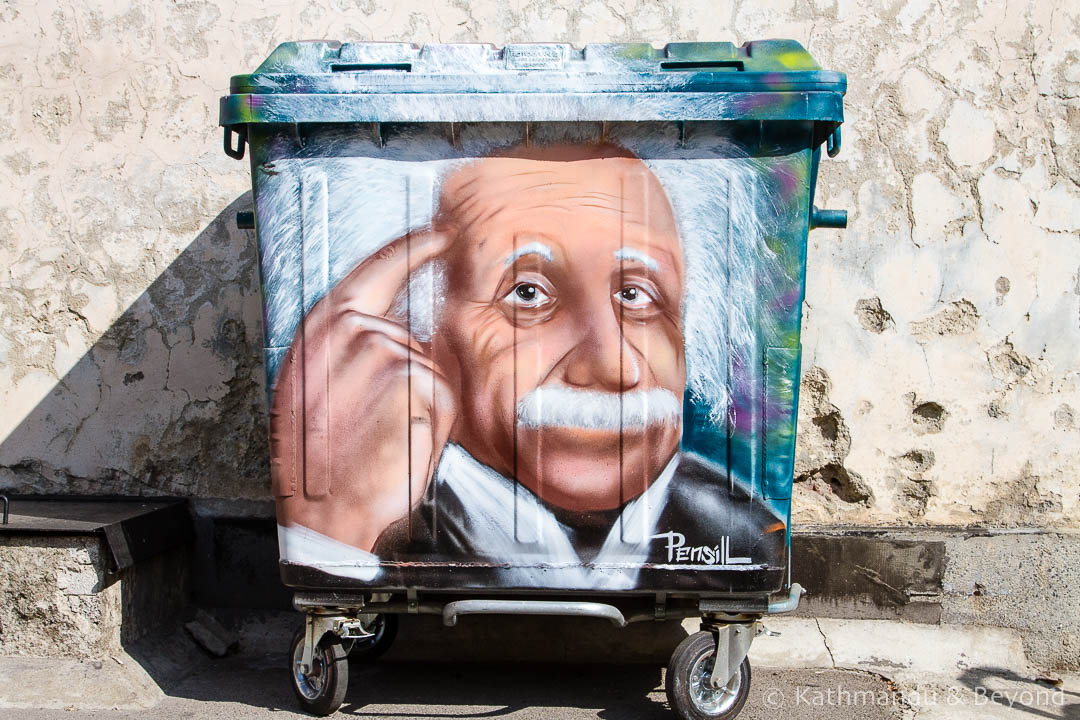This photograph, taken outdoors, depicts a wheeled trash can centered against a textured, plastered wall that shows signs of wear with gouges. The trash can itself, resembling a dumpster, is painted primarily in blue and green with accents of purple, tan, gray, black, white, peach, yellow, and various other colors. Prominently displayed on the front of the trash can is a cartoonish image of Albert Einstein’s head, characterized by his wild, white hair. Einstein's hand is raised with a finger pointing to his temple in a thinking pose while he looks straight ahead. Below this artwork, in the bottom right corner of the trash can, are the words "pencil" and a copyright attribution reading "Kath Manu and beyond." The lid of the bin is closed, and it's placed against a wall with a step visible to the left.